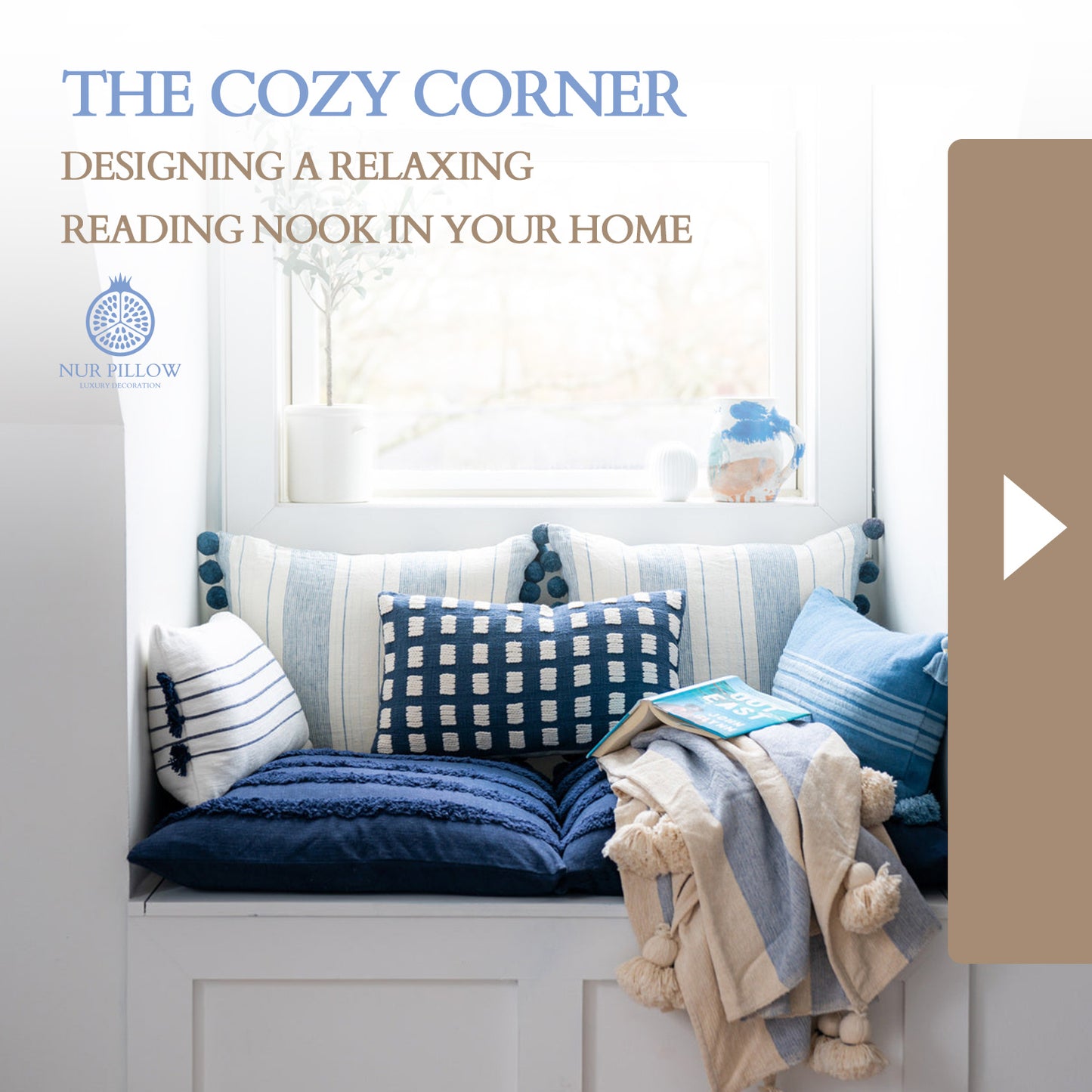This image is an advertisement featuring a cozy indoor reading nook. At the very top left corner, the text "THE COZY CORNER" appears in a light blue, all-caps font, followed below by "DESIGNING A RELAXING READING NOOK IN YOUR HOME" in a light brown, all-caps font. Just below this, a circular logo resembling the cross-section of an orange, accompanied by the brand name "NeuroPillow" in matching light blue, designates the product being advertised. 

The central focus of the image is a built-in bench seat nestled between white walls, positioned directly under a window. The bench is adorned with an assortment of pillows — a dark blue one, a light blue one, a blue and white striped one, and a checkered blue and white one. Laying across the blue cushions is a tan and blue striped blanket, atop which an open, light blue book rests. The window above the bench allows natural light to pour in, accentuating the cozy setup. On the windowsill, a small plant adds a touch of greenery, while a ceramic piece sits on the right side, enhancing the decorative ambiance.